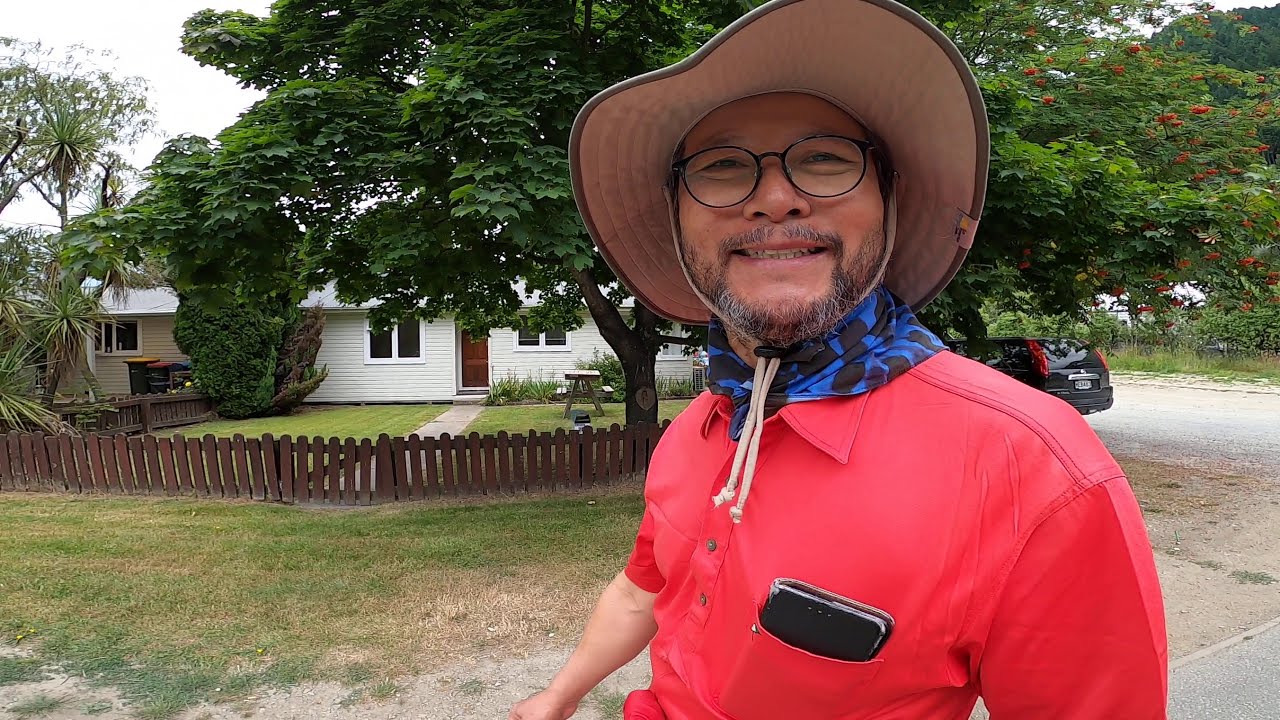A cheerful, older gentleman, perhaps of Hispanic descent, is walking on the sidewalk of a typical neighborhood street. He has a light graying beard and mustache and wears thin, wire-framed glasses. His attire includes a vibrant red button-down shirt with a cell phone tucked in the front-left pocket, and a blue and black patterned bandana around his neck. His head is adorned with a floppy field hat with strings under his chin. The man is smiling warmly, his eyes squinting slightly as he looks directly at the camera.

In the background, there is a well-manicured yard enclosed by a brown wooden picket fence. A white house with gray shingles and roof, flanked by bushes and trees, stands prominently. To the man's back right is a large tree with red flowers and, underneath it, the back half of a black Volvo station wagon is visible. The surrounding neighborhood features tropical trees, including palm trees, adding to the sunny daytime ambiance. The house has a path leading to its front door, highlighted by two windows on either side. Overall, this image captures a moment of everyday joy in a picturesque, peaceful neighborhood.